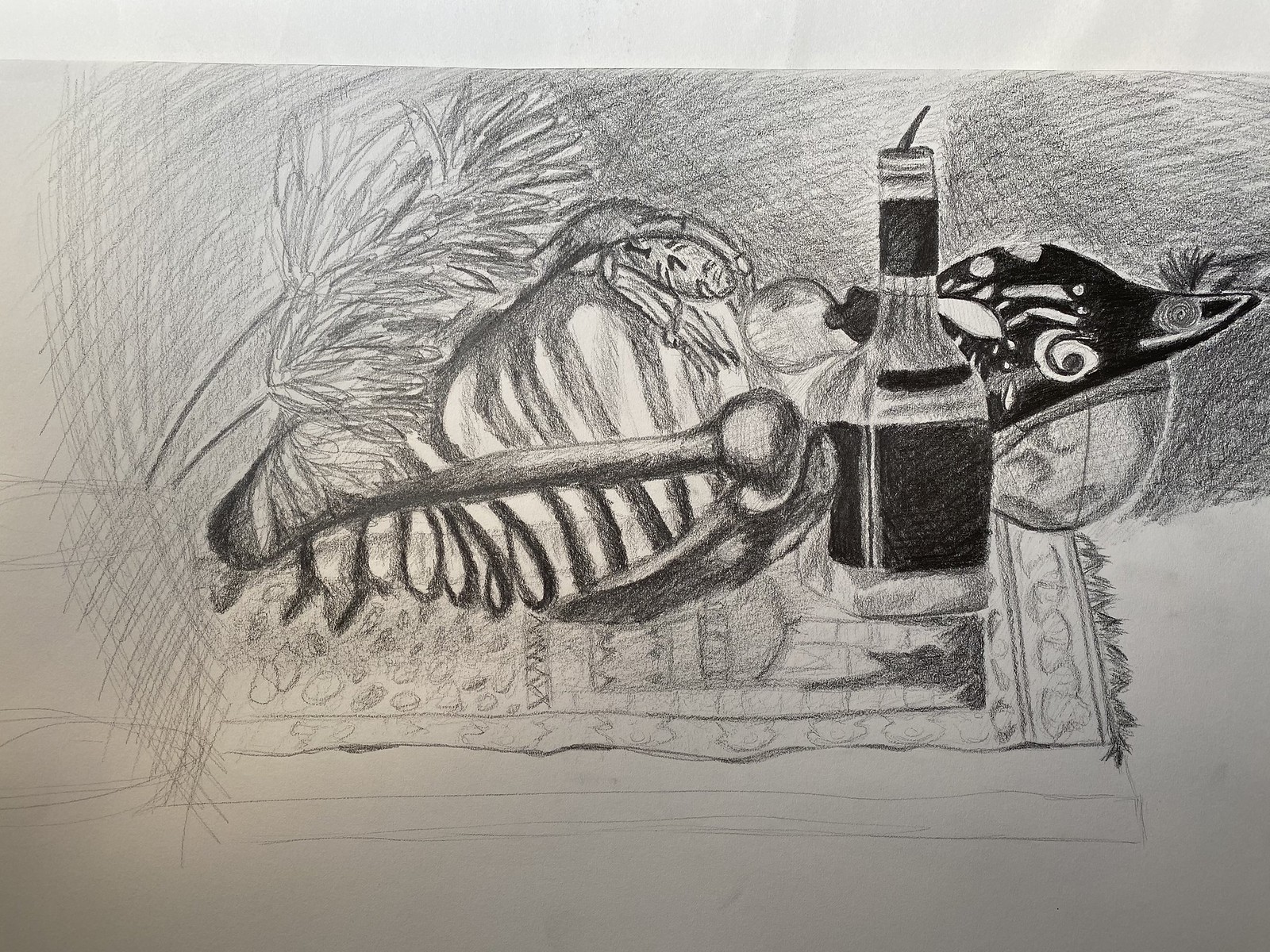This photograph captures a meticulously detailed pencil artwork, showcasing an intricately drawn still life. Executed in blended graphite, the composition features a pile of seemingly mismatched, yet captivating objects, purposefully arranged for a drawing exercise. The base of the arrangement is adorned with a detailed placemat, its intricate pattern evoking a burst of color despite the monochromatic medium. Dominating the composition is a tall, clear glass oil bottle, distinguished by a dark label that contrasts sharply with the surrounding elements. Adjacent to the bottle is a finely rendered, wood-carved loon head, its texture and contours flawlessly depicted. Sprigs of a delicate plant add an organic touch, complementing the scene with their intricate leaves and stems. Adding to the eclectic mix, a bone-like object is included, further enhancing the composition's intriguing diversity. Each element is sketched and blended with precision, showcasing the artist’s skill in capturing both detail and texture through the medium of pencil.